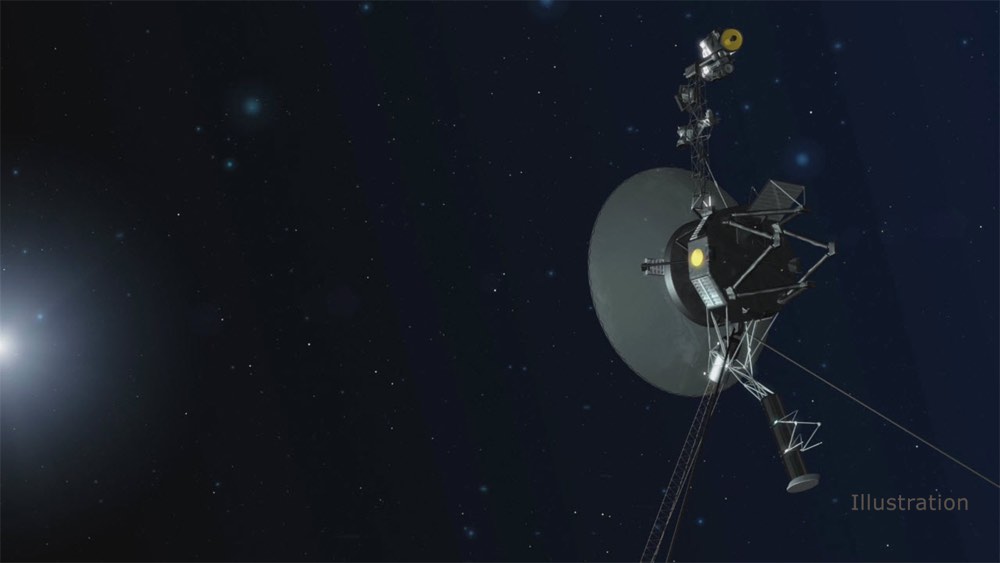This image depicts a dark, outer space scene with a navy-black background dotted with numerous tiny white star-like lights scattered throughout. The most notable feature on the left edge/middle-left edge is a bright white spot with a gradual white fade around it, which could represent the sun. Prominently situated on the right side of the image is a gray satellite. The satellite boasts a large gray dish facing left, topped with a yellow circle and accompanied by another yellow spot near the back. Various wires and bars extend from both the top and bottom, framing the structure. The word "illustration" is subtly inscribed in a sans serif font in the bottom right corner of the image.